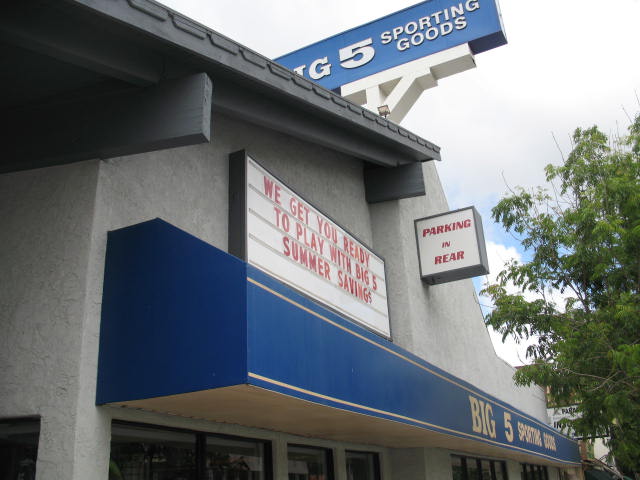The image showcases the storefront of a Big 5 Sporting Goods store. The building, made of gray stone, has a corner that is positioned about 20% from the left edge of the image. A dark blue awning with gold lettering reading "Big 5 Sporting Goods" juts out prominently from the right side of the building. Below the awning, there are double doors that appear closed and somewhat dark, hinting at a gloomy interior. A prominent sign above the entrance reads, "We get you ready to play with Big 5 Summer Savings." There is also a smaller red sign indicating "Parking in Rear" that's protruding from the building. The gray stucco building, reminiscent of 1980s architecture with its slanted wooden roof, extends into the distance on the right side, where a tree can also be seen.